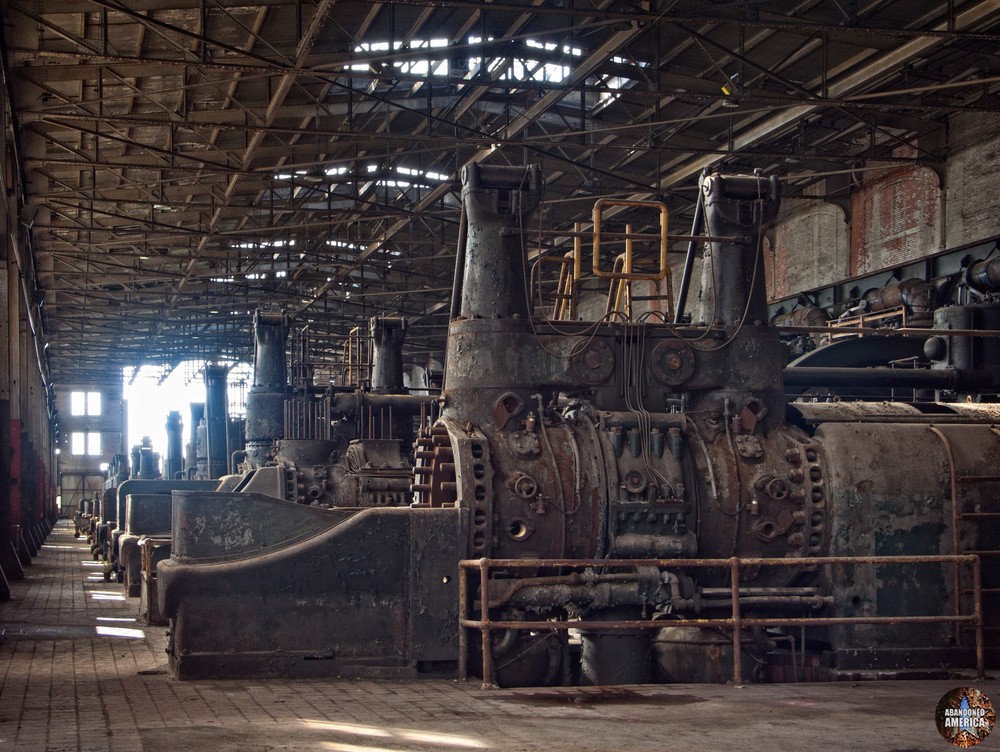The image depicts a row of abandoned, intricately detailed railway engines positioned under a large, dilapidated industrial structure with a high, steel, grid-like roof, showing signs of rust and age. The engines, steeped in a brown and gray palette of rust and decay, are connected by a network of cables and piping, revealing a history of heavy use and neglect. They span the length of the floor, which is composed of worn wooden planks or brick pavers, each with vertical slats and joints visible, contributing to the derelict atmosphere. The space is adorned with a complex web of steel tubes, iron beams, and metallic fixtures, including valve handles, bolts, and rivets, indicative of industrial machinery such as turbines or generators. The floor shows additional signs of degradation with rusted bars and a dingy, grimy surface. The deteriorating roof, with its metallic framework and sporadic holes, allows beams of light to penetrate, illuminating the scene with a stark, eerie quality. On the right side of the image, there is a brown circular logo with a star inscription reading “Abandoned America,” reinforcing the theme of forsaken industrial grandeur. The building’s exit is discernible towards the left center, and the overall impression is one of haunting desolation and mechanical remnants of a bygone era.